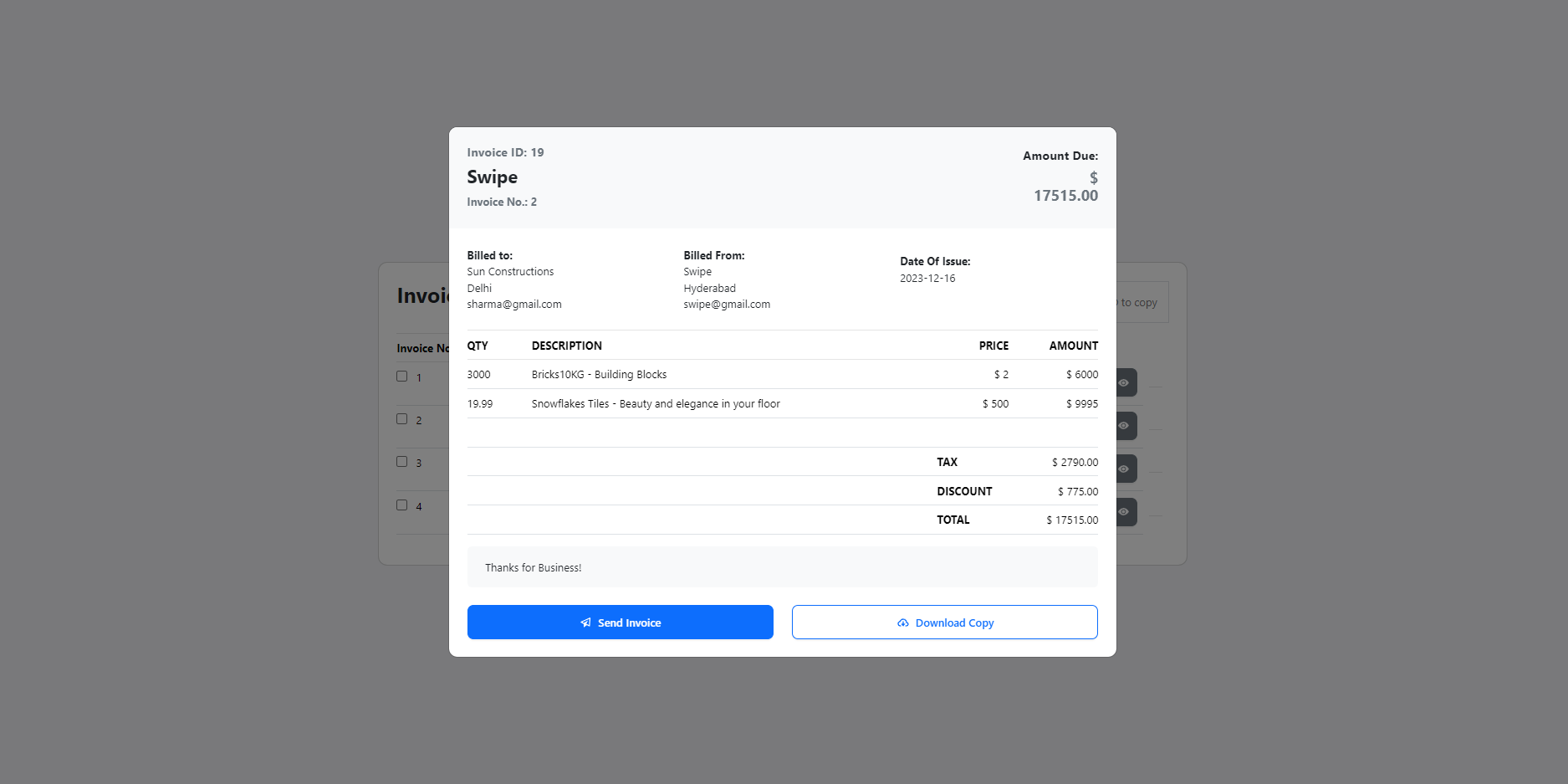This image is a screenshot of a digital invoice displayed on a website. In the center of the image, there is a prominent white square with the instruction "Swipe" written on it. In the upper left-hand corner, there is small text indicating "Service Number: 2." Below this, in a slightly larger font, the amount due is stated as "$7,513.00."

Inside the white square, further information is presented in very small, almost illegible print. It includes the "Bill to" address, which appears to be labeled "Build" or something similar. Additionally, there is a date—likely the purchase or installation date—though it's difficult to read.

The description section lists items or tools purchased, along with their corresponding prices and amounts. Taxes, discounts, and the total amount due are clearly outlined. 

On the right-hand side of this section, there's supplementary information. On the left side, under the main content, there's a possibly unclear text, concluded with the phrase "really again." Below this, a blue bar with white writing runs across, beside which is another white bar that contains the word "Download" in blue lettering.

Overall, the document appears to be an itemized digital invoice with detailed purchasing information, amounts, and specific financial and billing details.